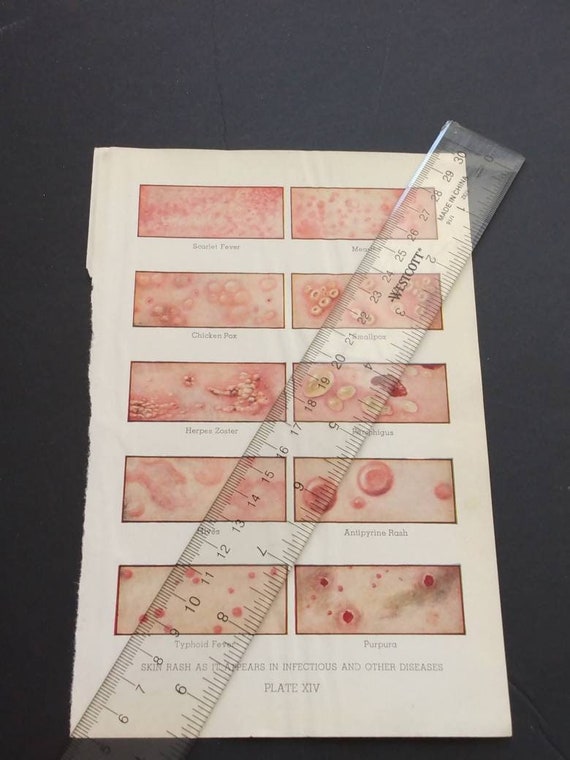The image depicts a cream or off-white page from a book, possibly a textbook, laid on a dark gray or black surface. The page features detailed illustrations of various skin rashes and irritations, arranged in two columns and five rows of horizontal rectangular images. Each illustration predominantly features different shades of pink with round and irregularly shaped lesions. Beneath each image, there are captions identifying conditions such as scarlet fever, chicken pox, smallpox, herpes, rash, and typhoid fever in dark or gray text. At the bottom of the page, there is a caption in gray text that reads, "Skin rash as it appears in infectious and other diseases, plate XIV." A clear, transparent ruler lies diagonally across the page, stretching from the bottom left to the upper right corner, partially overlaying the illustrations. The ruler displays measurements in centimeters from 6 to 30 on the top edge and from 0 to 9 on the bottom edge. The top right corner of the ruler bears the inscription "Westcott made in China."